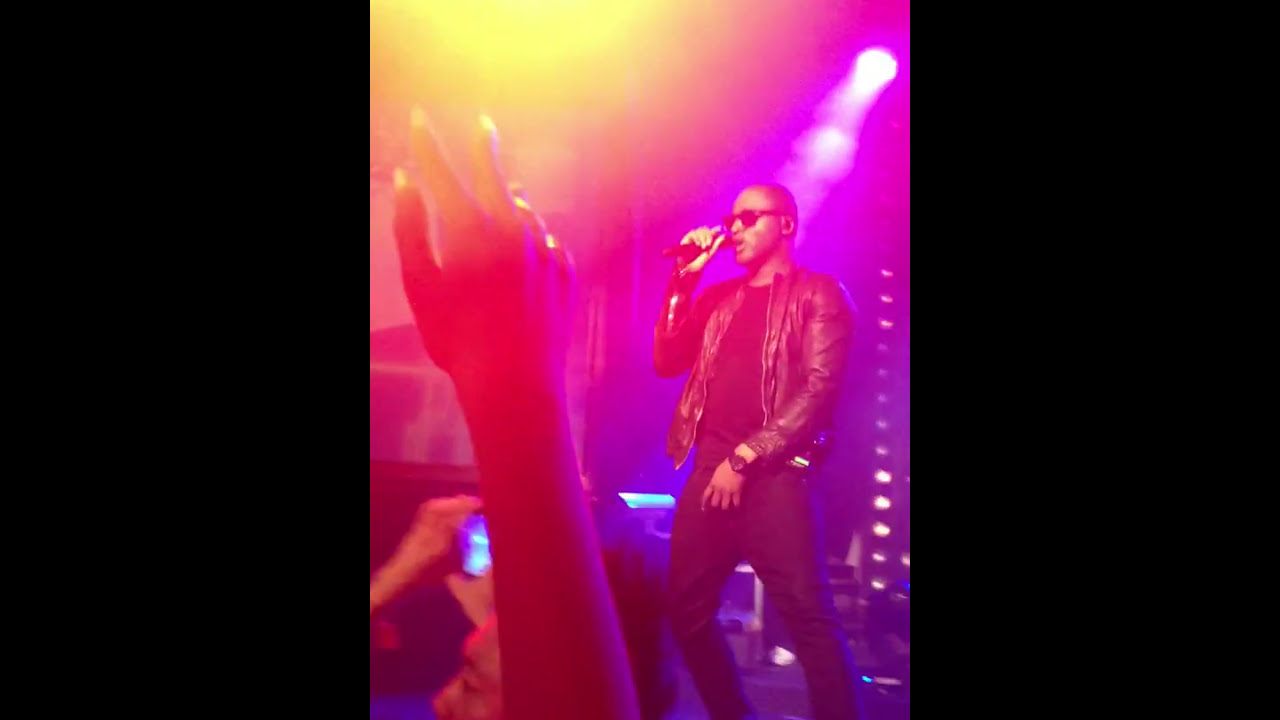In this vivid indoor photograph, set in the dynamic environment of what appears to be a nightclub or concert hall, a young black man is captured mid-performance, singing into a microphone with a passionate intensity. His attire consists of a striking red leather jacket, black pants, and a black t-shirt, complemented by stylish sunglasses. The energetic scene is brought to life under the glow of two spotlights illuminating his head from behind, adding depth to the predominantly pinkish-purple backdrop. Additionally, an orange spotlight in the upper left-hand corner adds a dramatic flair. 

Prominently in the foreground, the raised arm of a spectator—hand with three fingers extended—acknowledges the singer, enhancing the sense of connection between performer and audience. The edge of another spectator's face and hair is visible next to the arm, indicating a crowded, lively audience deeply engaged with the performance. The entire photograph, framed as the center panel of a three-panel layout with black rectangles flanking either side, encapsulates the vibrant atmosphere of the concert and the palpable energy of the moment.